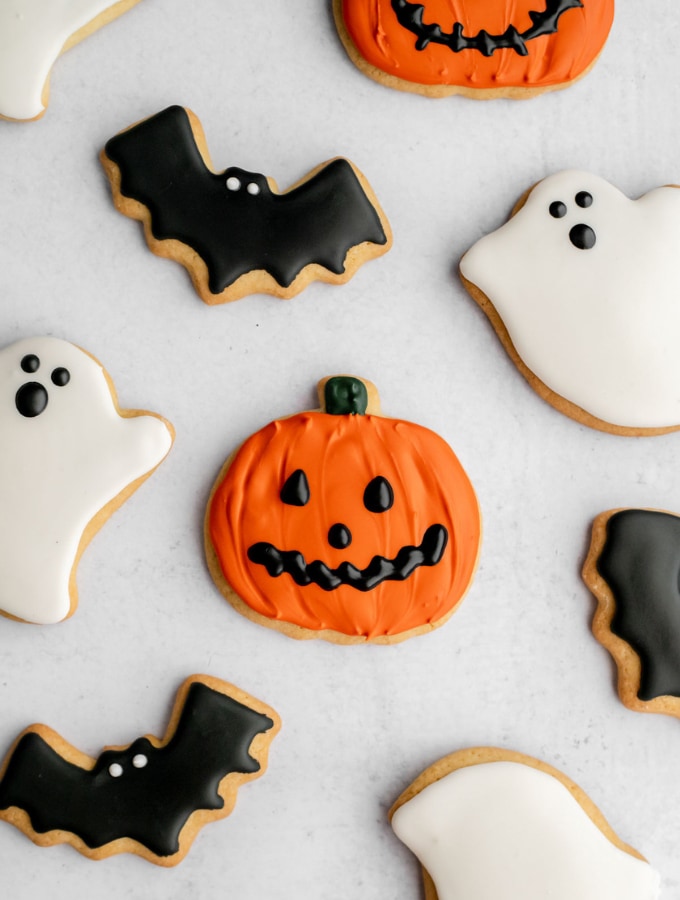This image vividly captures an array of Halloween-themed sugar cookies, meticulously decorated and arranged on a light-colored stone countertop speckled with darker elements. The cookies, cut into festive shapes, span the entire frame, some extending beyond its edges. At the top of the image, a partially visible pumpkin cookie with orange frosting and a green-stem detail adds a splash of color. The centerpiece is another pumpkin cookie, prominently displayed with black icing forming expressive eyes, a small nose, and a squiggly mouth. Surrounding the pumpkins are three bat-shaped cookies, each adorned with smooth black frosting and marked with tiny white dots for eyes, although one bat is only partially visible. The scene is further complemented by four ghost-shaped cookies, two of which are mostly visible, flaunting white frosting with simple black dots for eyes and slightly larger black dots for mouths. Each cookie, crafted from a beige sugar dough, exudes a charmingly eerie holiday spirit through its meticulous icing details.